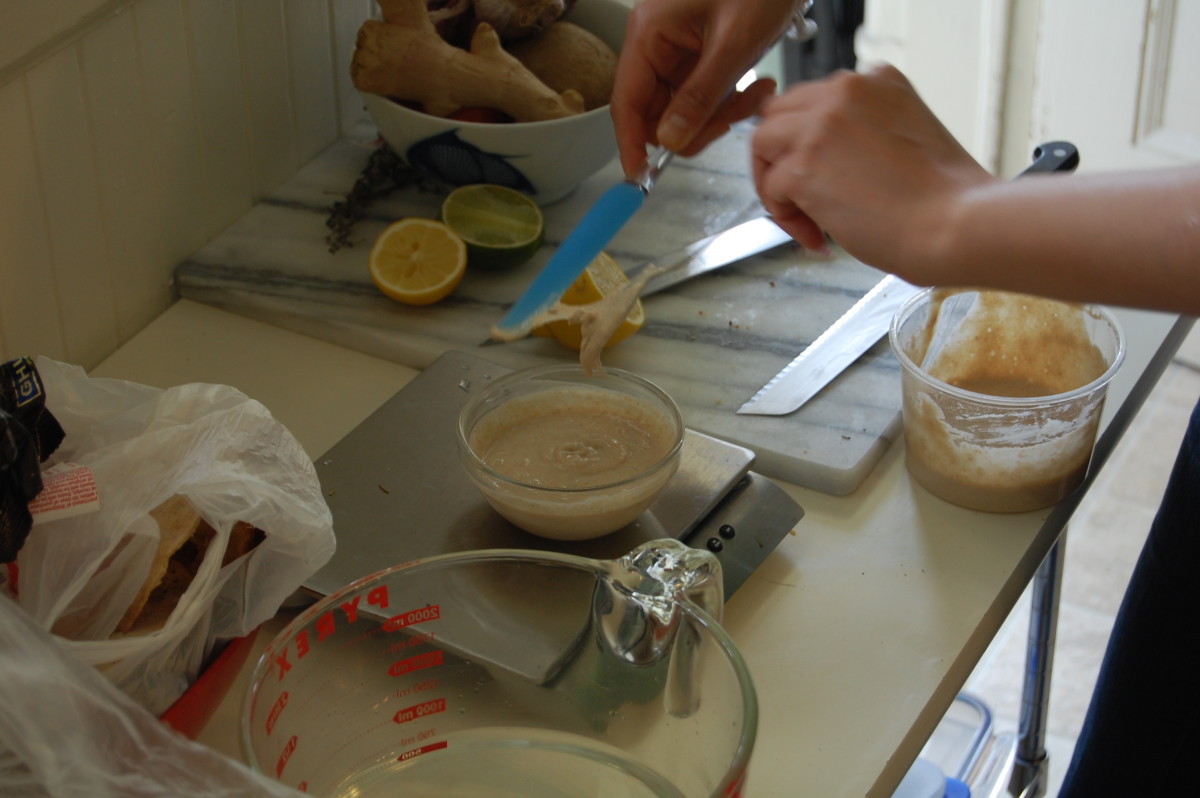In this detailed kitchen scene, a Caucasian individual is meticulously preparing an ingredient using a unique knife with a silver handle and a distinctive blue blade. They are seen extracting sauce from a bowl and carefully measuring it on a gleaming silver weight scale. To the left of this person, a glass measuring jug featuring red measurement markings stands near a clear plastic bag positioned above it. On the right side of the setup, there is a sharp silver knife with a black handle and a clear jar containing a brown paste. The individual works on a small off-white table, which features a cutting board with white and black marble-like patterns. On this cutting board, there is a halved yellow lemon and a whole green lime beside it. A white bowl located at the top right holds what appears to be pieces of yellow ginger. The backdrop is composed of off-white tiles, and underneath the table, a clear blue-lined plastic container can be seen. A white door is positioned at the top right, completing the kitchen's layout.